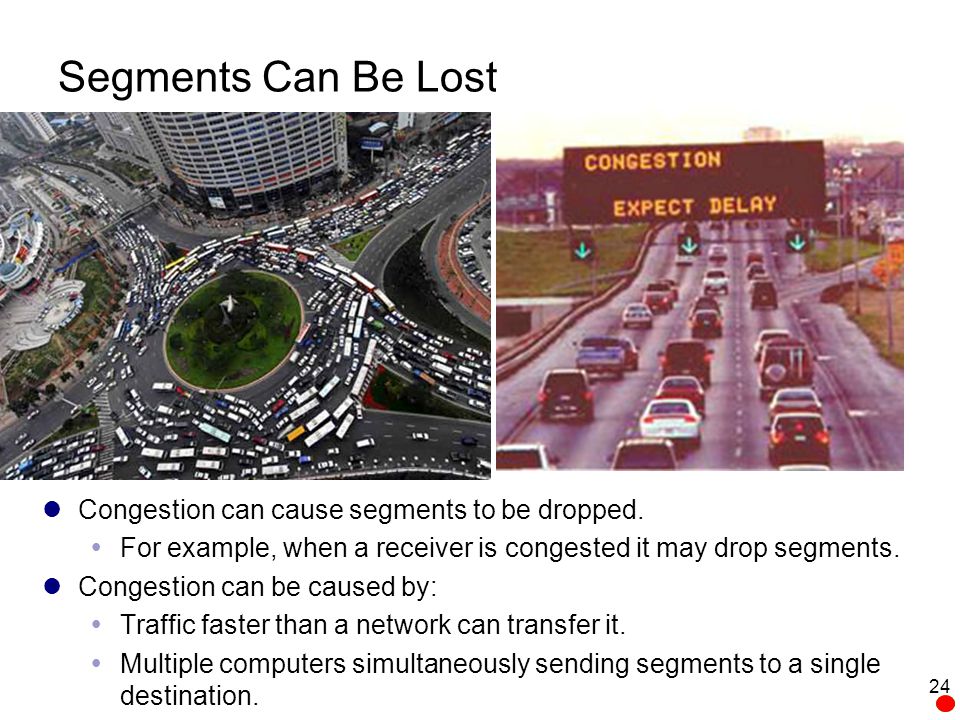The educational slide features two primary images depicting traffic congestion. On the left, there is a roundabout swarming with cars caught in a gridlock, emphasizing the difficulties of navigating heavy traffic. The right side shows a busy multi-lane highway with an overhead digital sign displaying "Congestion, Expect Delay" in orange. Both images illustrate the concept of network congestion and its impact on data transmission.

The slide includes detailed explanatory text. At the top left, it states, "Segments can be lost." Below the images, bullet points elaborate on how congestion can cause segments to be dropped, noting that, for example, when a receiver is congested, it may drop segments. It further explains that congestion arises from traffic outpacing the network's capacity and multiple computers sending segments to a single destination simultaneously.

The slide's color scheme features a mix of gray, red, black, white, green, blue, and orange, enhancing its visual emphasis on traffic scenarios and technical points. Additionally, there's a notable red dot with the number 24 above it, positioned subtly within the scene. This detailed educational graphic effectively merges visual and textual elements to convey the impact of congestion on data networks.